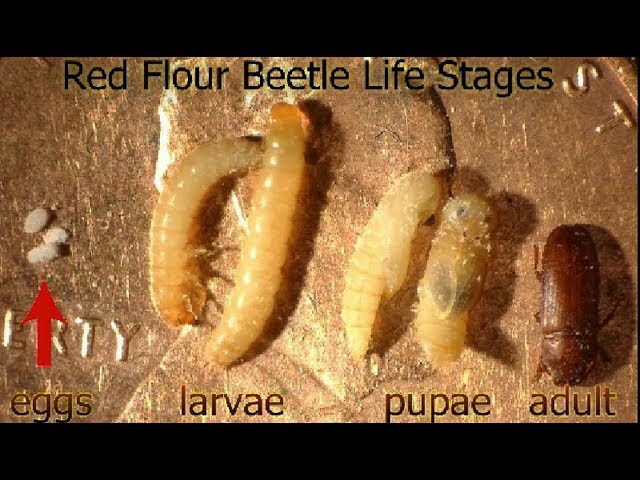The image is entitled "Red Flower Beetle Life Stages," displayed in black letters across the top. Below the title, the four life stages of the red flower beetle are illustrated in sequence from left to right. The first section, labeled "eggs" at the bottom, shows three small, white, oval-shaped eggs with a red arrow pointing up to them. Next, the "larvae" stage is depicted with two worm-like grubs that are pale beige or light yellowish in color, each with visible tiny feet. Following that, the "pupae" stage is shown, with two shorter, plumper, and paler grub-like forms, representing the early development of the beetle. Finally, the "adult" stage features a red-brown beetle with distinct legs visible at both the front and back, labeled "adult" at the bottom. The beetle depicted appears somewhat similar to a cockroach in shape.